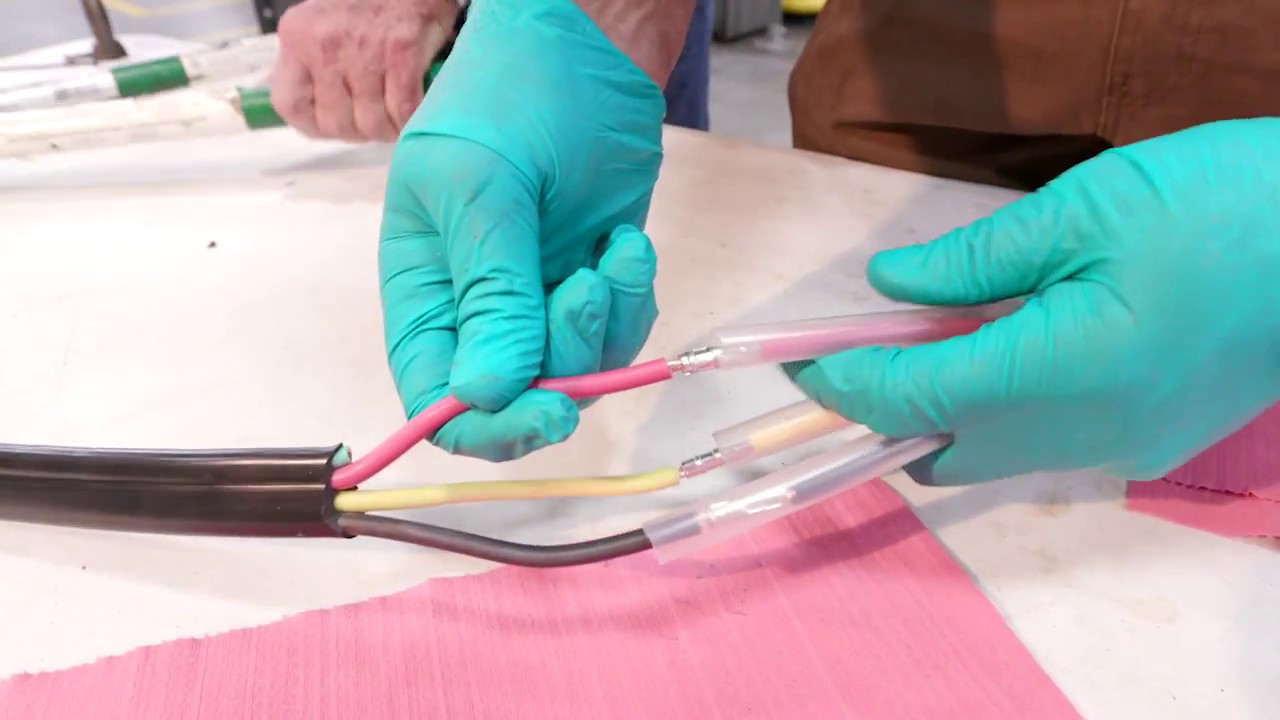This close-up photograph captures a meticulous setup where a person, wearing greenish-blue surgical gloves, works over a clean, white surface. In the bottom left corner, a large black tube extends to the right and slightly downward before splitting into four smaller tubes: a pink one going upward left, held by a gloved hand; a yellow one running up right into another gloved hand; another yellow tube going straight into a plastic tube; and a black or dark tube curving downward then upward into another plastic tube. Both gloved hands are centrally positioned—one descending from the middle top, holding the pink tube between the thumb and forefinger, guiding it toward another plastic tube, while the other gloved hand, emerging from the right side above the center, secures the other tubes between its fingers. A pink rectangular cloth rests on the white tabletop at the image's bottom. In the image's upper left, an ungloved hand—presumably another person's—enters from the top, showing only a partial view of a bare wrist and bent knuckles beside a set of glass or plastic tubes with green bands. The upper right reveals a hint of brown, likely clothing of the glove-wearing individual. The dynamic arrangement of tools and hands suggests a detailed and precise task, possibly related to wiring or medical work involving tubing and cables.